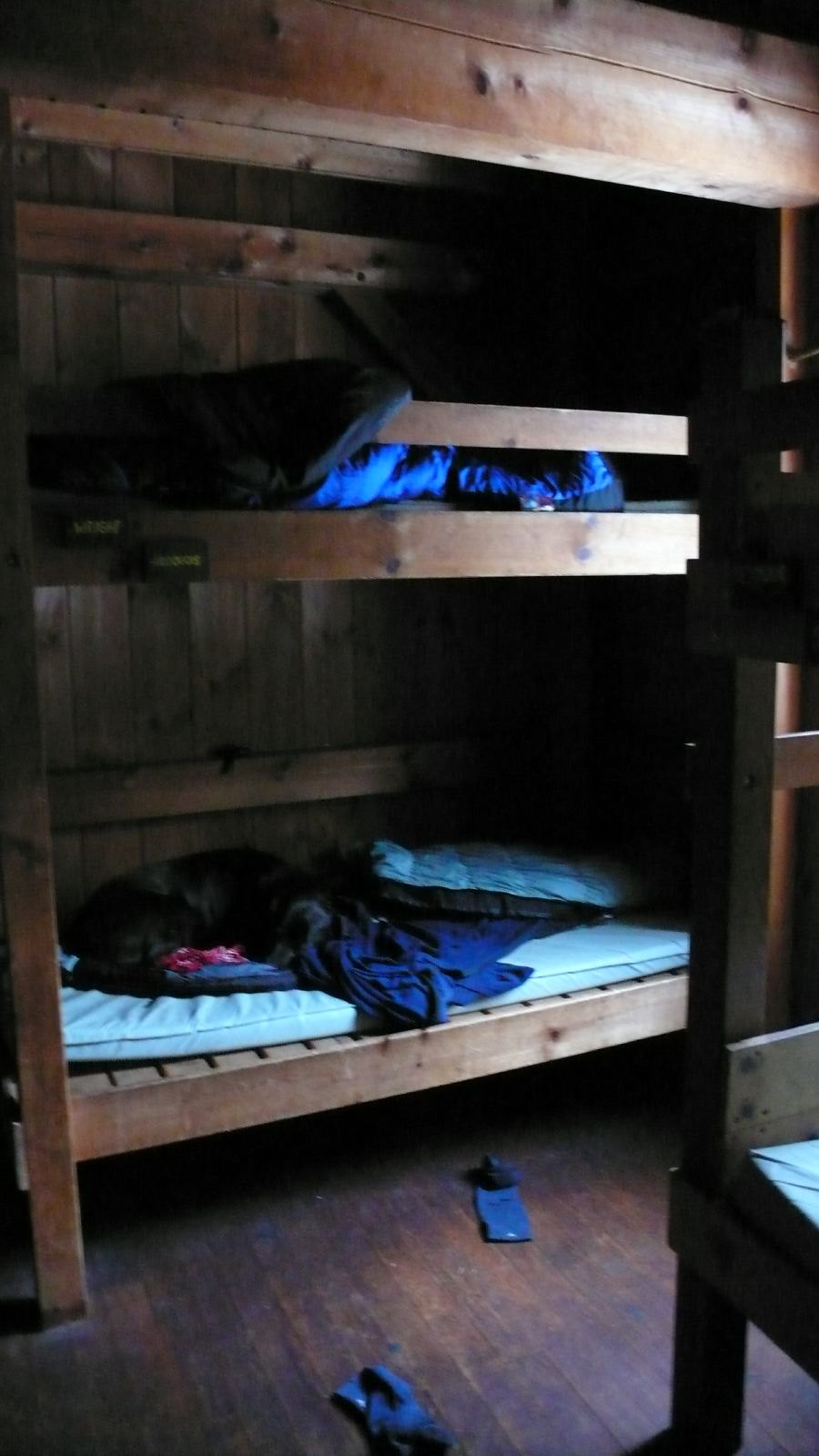The photograph captures the interior of a wooden cabin, with dark wooden floors and wooden panels on the walls, evoking the rustic simplicity of a summer camp setting. Dominating the composition are two basic wooden bunk beds, built into the structure. The lower bunk is equipped with an incredibly thin, light aqua blue mattress, and is currently occupied by a black Labrador sleeping soundly. Scattered at the bottom of the bunk are blue socks or slippers, and a blue vest lies atop the mattress next to a matching blanket. The upper bunk is minimalist, featuring a small protective rail and what appears to be either a blue sleeping blanket or possibly a black blanket draped over the edge. Attached to this bunk are two square name tags with indistinct writing. The room is modestly lit, creating a contrast between patches of light and the generally darker ambiance. To the right, partially cropped by the image frame, another bunk bed is hinted at, its vertical posts and segments of the top frame and mattress visible. The overall scene lacks personal effects, and the sparse furnishings further suggest the temporary, utilitarian nature of a holiday camp dwelling.